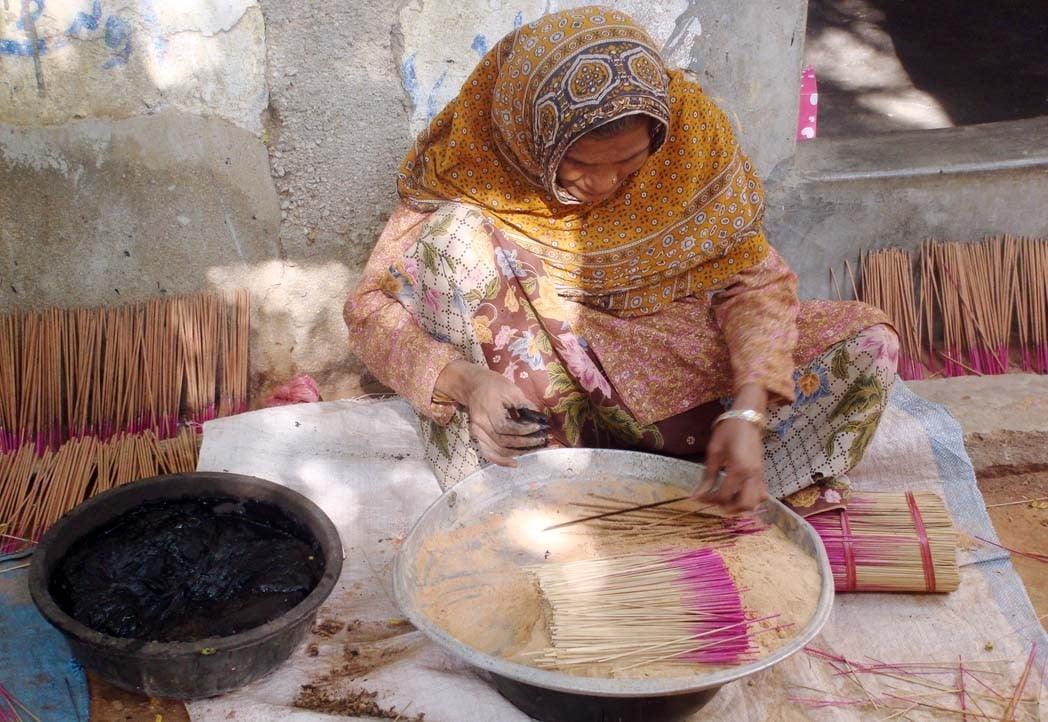A woman is leaning against a large concrete wall adorned with small blue markings, sitting on an off-white mat with bamboo sticks beneath her feet. She is dressed in an orange-gray patterned outfit featuring pink patterns and squares on what would be the skirt area. To her left is a gray bowl containing a black substance. In front of her, there is another large gray bowl filled with brown powder, topped with gray and pink sticks. She wears a silver bracelet on her left wrist and holds one of the gray sticks with a pink tip. There are two stacks of items to her left and one stack to her right, positioned near a gray ledge that leads into a darker area to her right. The ground beneath her is predominantly brown on the bottom right side, with a blue object visible at the bottom left.